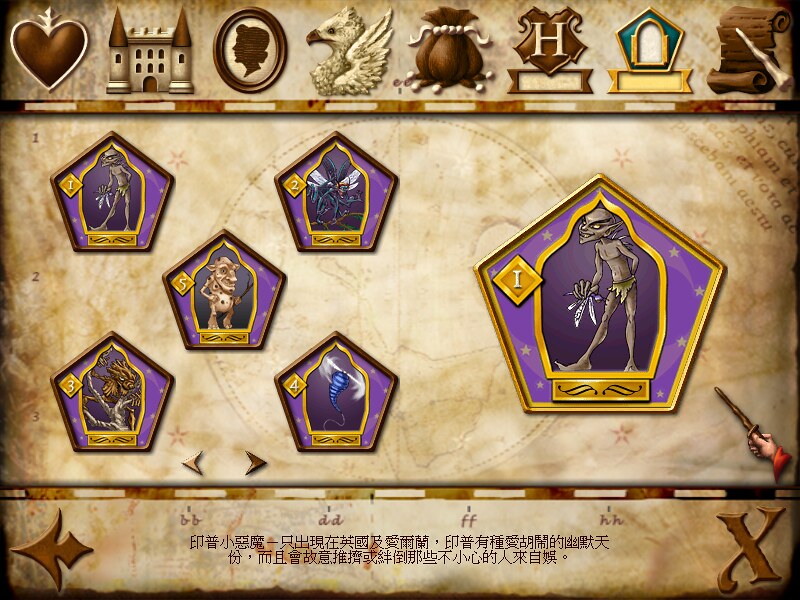The image depicts a menu screen from a fantasy video game, potentially influenced by Harry Potter, featuring a brown parchment-like background with splotches, reminiscent of a treasure map or the Muggle map. At the top, a series of icons likely used in the game are displayed, including a heart, a castle, a cameo of a woman's head, a phoenix, a treasure satchel, a family crest with an 'H', a doorway resembling the one under Harry Potter's stairs, and a parchment with a wand. Central to the screen are six pentagonal badges, five small ones and one larger, each showcasing different monsters highlighted with purple and gold colors. These badges appear interactive and selectable, possibly representing different levels or lands in the game. The user can seemingly navigate these options using a small hand image holding a magic wand in the bottom right corner. Chinese writing is present at the bottom of the screen, further hinting at the game's global or diverse setting. Navigation arrows are situated at the bottom right and left corners of the screen, completing the interactive menu layout.